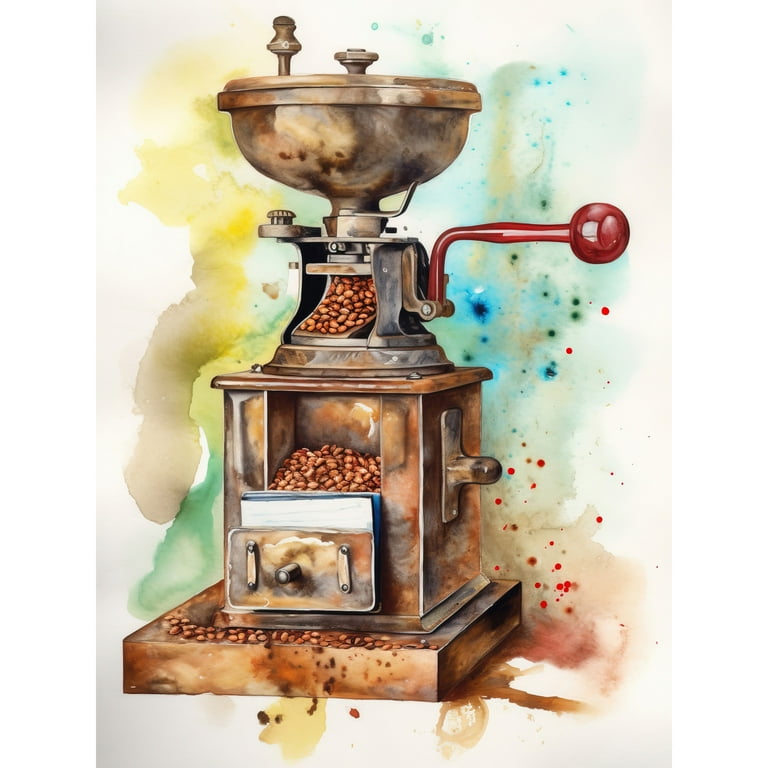The image is a detailed watercolor painting of a coffee grinder, rendered in a mix of brown and gray tones representing its primarily metal construction. The grinder features a square base with a metal drawer slightly open, revealing brown coffee beans. Its central body is rectangular, leading up to a round bowl at the top, also filled with coffee beans. A distinctive red handle with a red ball tip extends from the side, which appears to be a crank or latch. The background is an abstract blend of watercolor splotches and drips in yellow, blue, green, and red, adding a vibrant, runny color effect around the realistically painted coffee grinder. The overall artwork gives a sense of a traditional, vintage coffee grinder through the medium of expressive, colorful watercolor painting.